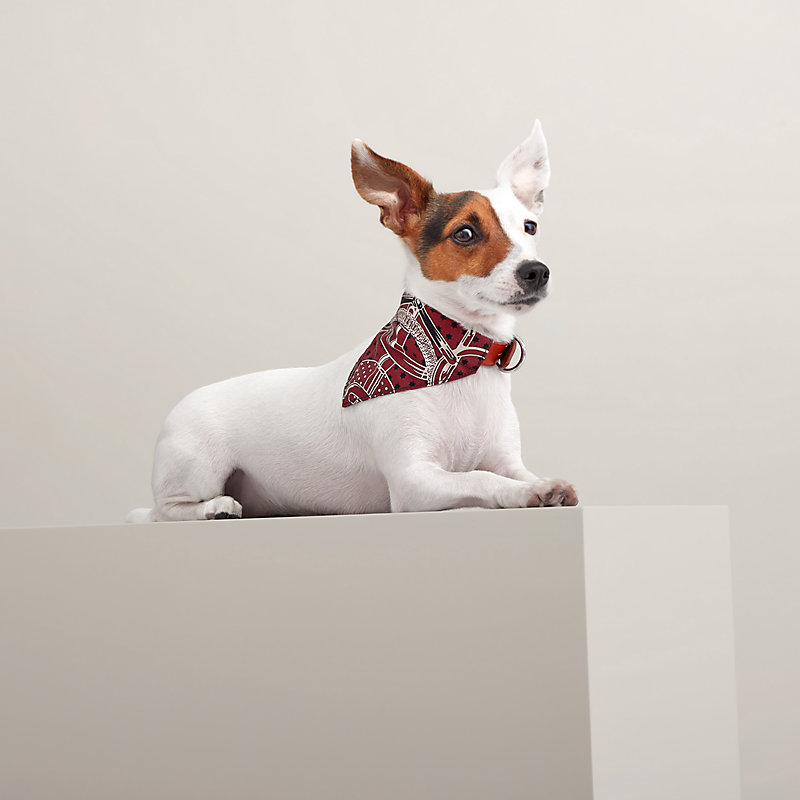This image features a close-up of a small, smooth-haired terrier sitting atop a white cube against a grey background, likely from a photoshoot. The terrier is predominantly white, except for its right eye and ear, which are brown with hints of maroon, giving it a distinct two-toned face. Its black nose and expressive black eyes stand out, as do its upright ears. The terrier's paws are positioned at the front edge of the cube, with its right hind leg visible. Around its neck, it wears a collar with a red leather design and an attached triangular bandana that extends down to mid-body, featuring white and black patterns. The dog is gazing directly at the camera with its mouth closed, exuding a poised and composed demeanor.